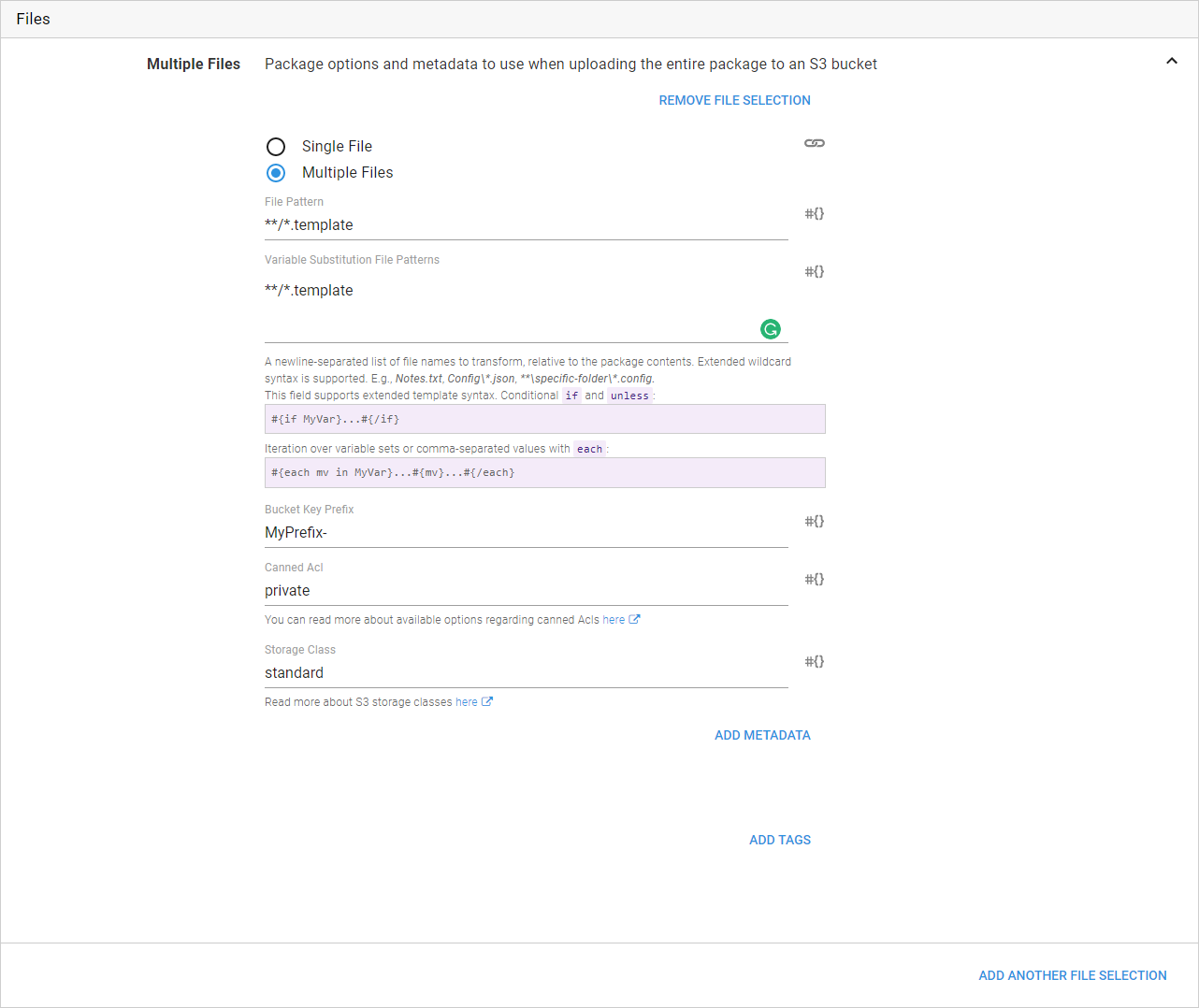The image captures a software interface titled "Files," displayed in a light purple-gray bar across the top. Below the title, bold black text states "Multiple files," with accompanying metadata options for uploading files to an S3 bucket, titled "Package Options." Beneath this, a blue hyperlink reads "Remove file selection." 

Two file selection options are presented: "Single file" and "Multiple files," with the latter being selected. Fields labeled "File Pattern Template" and "Variable Substitution File Patterns Template" describe a new line-separated list of file names for transformation relative to the package contents, supporting extended wildcard syntax. Notes mention the configuration of JSON-specific folder settings, extending support for template syntax using conditional statements such as "if" and "unless."

Two code entry boxes are present, labeled "My Prefix" and an option indicated as "Private." Users are also provided a link to "read more about available options." Lastly, the storage class is set to "Standard."